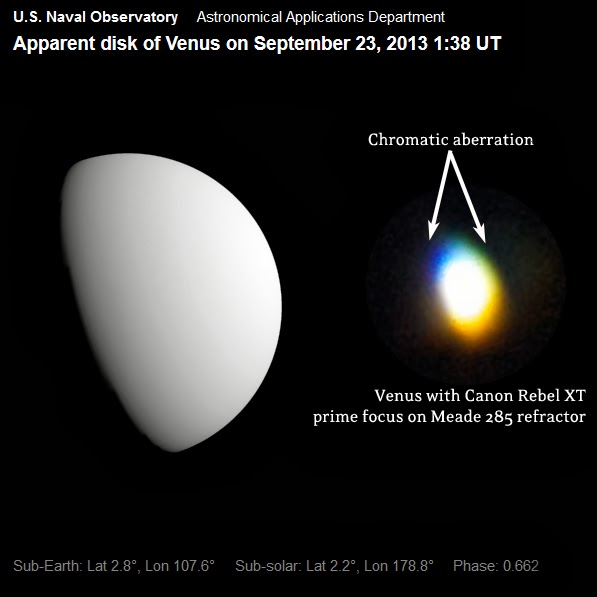This is a detailed poster set against a black backdrop, titled "U.S. Naval Observatory, Astronomical Applications Department." Dominating the image is a solid white disk representing Venus on September 23, 2013, at 1:38 UT. The disk appears to fade at the bottom into the black background. Notably, the poster highlights a chromatic aberration effect, depicted with multi-colored hues and linked by white arrows to an image described as a "fiery ball." The text details that the image of Venus was captured using a Canon Rebel XT camera, with prime focus on a Meade 285 refractor. The bottom of the poster provides specific astronomical coordinates and data, including sub-Earth and sub-solar latitude and longitude, as well as the phase number of Venus. This intricate information would likely be appreciated by those with a background in astronomy.